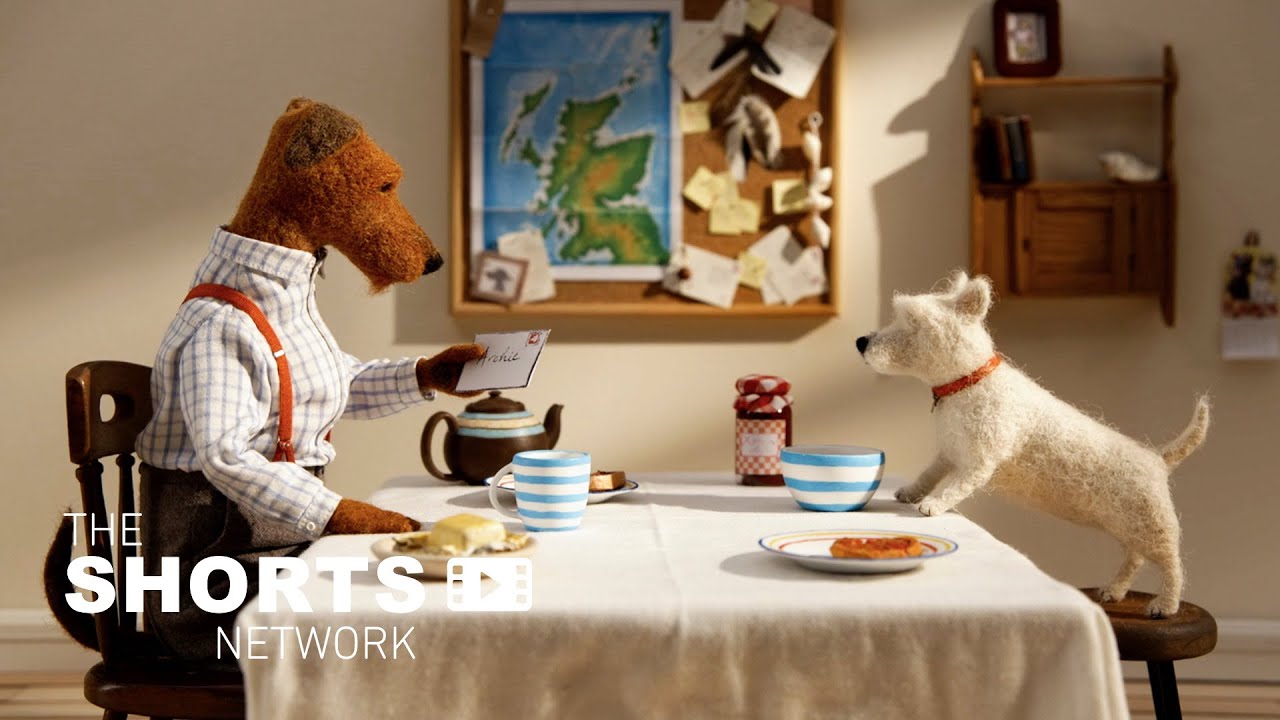This is a promotional photo for the children's TV show, The Shorts Network. The image captures a cozy kitchen scene featuring two plush dog figures at either side of a table draped with a white tablecloth. On the left, a small, realistic-looking white dog with a red collar stands on a brown stool, balancing himself with his front paws on the table. Across from him, a much larger plush dog with ginger-colored curly fur sits upright on a wooden chair. The larger dog is dressed in a checkered button-up shirt with white and blue squares, orange suspenders, and brown pants, holding a white piece of paper in his left paw as if he is showing it to the smaller dog. 

The table is set with blue-and-white striped mugs and bowls, a tea kettle, and plates with food, possibly toast and jelly. A map and a shelf can be seen in the background, adding to the homey atmosphere. The overall scene suggests a playful, engaging moment between the two character figures, ideal for a children's show setting.